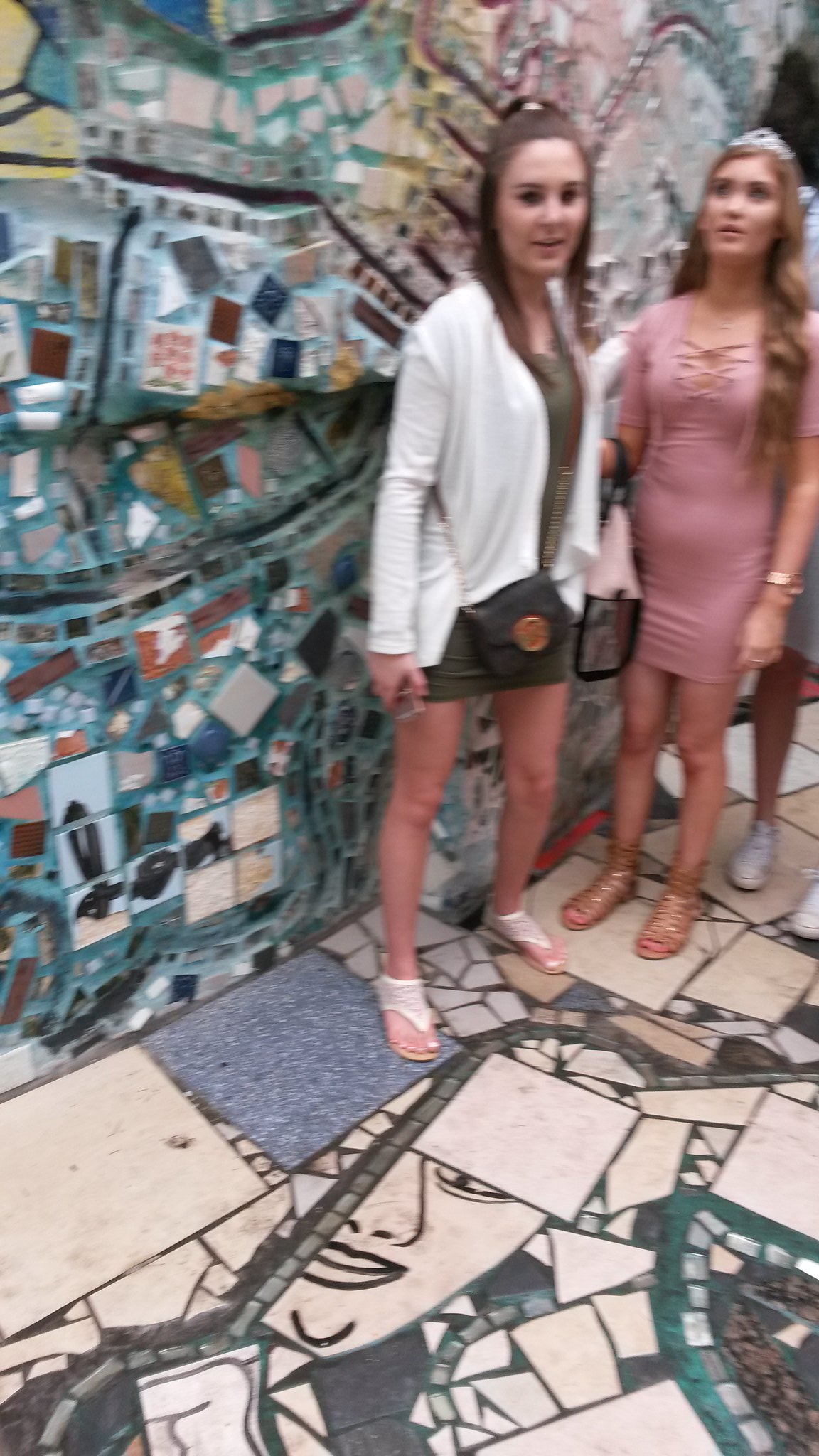In this image, we see two teenage girls posing in front of the vibrant and artistic stained-glass exhibition in Philadelphia. The background features a colorful mosaic wall composed of various shapes and hues, especially teal, turquoise, black, and white. The floor beneath the girls is equally intricate, designed with multi-colored stone tiles forming faces and abstract patterns.

The girl on the left is wearing a short green dress paired with a white sweater and holding a green purse. She has medium-length brown hair and a slight smile, staring directly at the camera. The girl on the right is adorned in a pink dress and a silver tiara, with long brown hair cascading down her shoulders. Both girls appear to be engrossed in capturing the beauty of the exhibit, while a third person, only partially visible with white tennis shoes, stands behind them.

The image is slightly blurry, adding an element of spontaneity to the moment captured, but it doesn’t overshadow the detailed and rich mosaic artwork that adorns both the floor and the wall, creating a visually captivating scene.